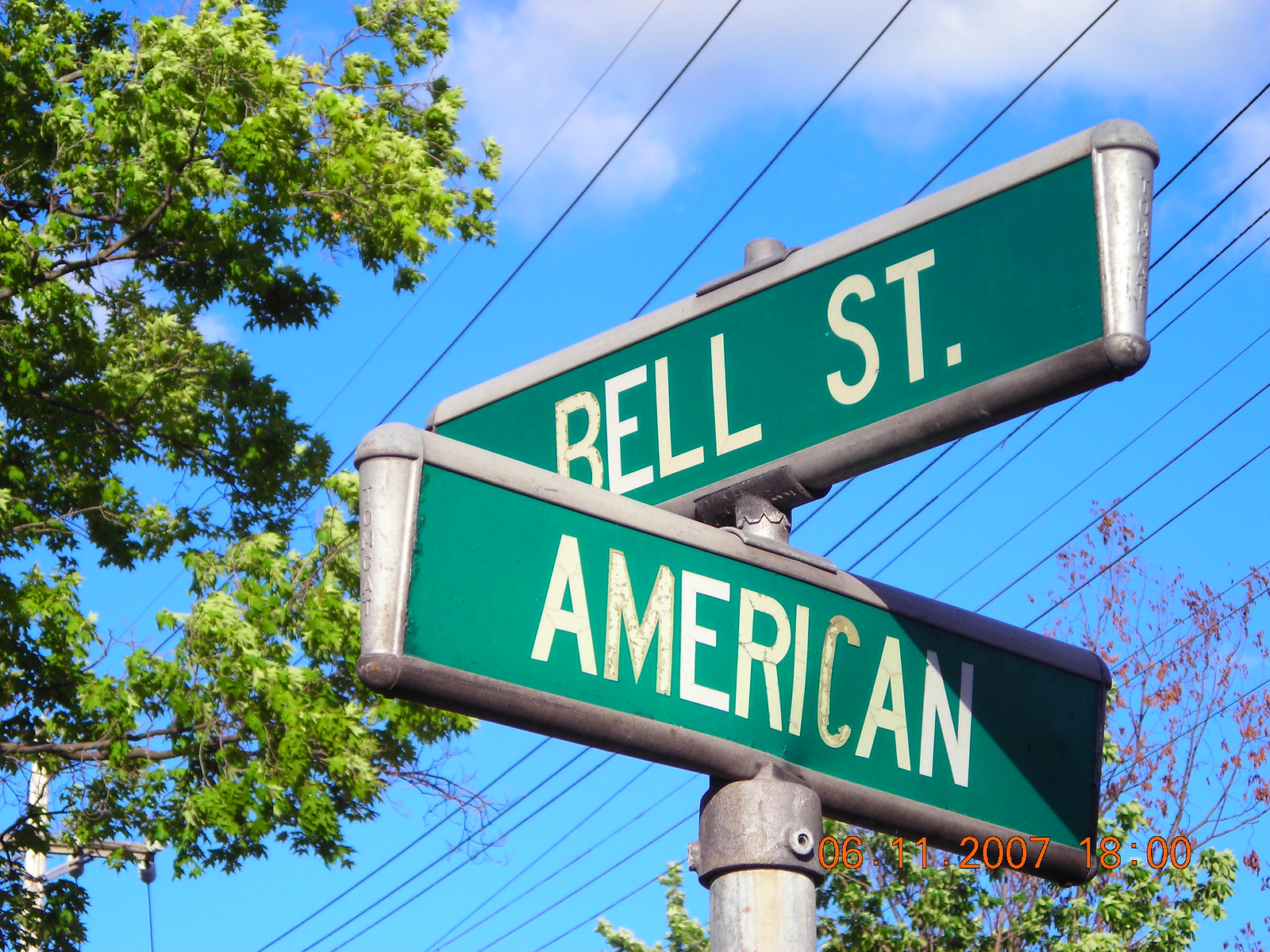The image showcases two intersecting green street signs mounted on a gray pole. The top sign reads "Bell St." in bold white letters, with silver borders on the top and bottom. Below it, another green sign displays "American" in similar white letters, also bordered in silver. Both signs are connected by brackets to the pole.

Surrounding the signs are two vibrant green trees, one positioned to the left and another to the right. Additionally, a distinctive pink tree stands on the right side, adding a pop of color to the scene. Power lines run horizontally across the background, contributing to the urban setting. In the bottom right corner of the image, a timestamp reads "06-11-2007-1800," indicating the date and time the photo was captured.